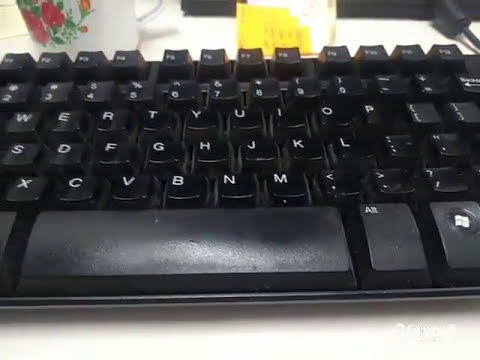A detailed image of a traditional black computer keyboard with white lettering, featuring common keys such as the Windows emblem key, a wide space bar, and the Alt key. The keyboard layout is slightly unconventional as it starts with the letter 'W' instead of 'Q' for a QWERTY layout, showing the sequence: W, E, R, T, Y, U, I, O, P on the top row and S, D, F, G, H, J, K, L on the row below. The bottom row includes X, C, V, B, N, M keys. The keyboard is positioned on an off-white counter with yellow post-it notes and a white mug decorated with an image of red roses with green leaves placed to the left. Behind the post-it notes, part of a monitor or another computer device is visible, marked by a black bar. The keyboard appears clean, and its front end shows a cash saddle.